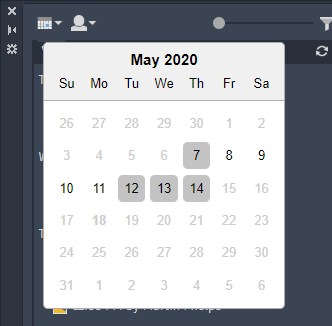A screenshot displays a calendar application in a pop-up window with a white background. At the top of the calendar, "May 2020" is prominently displayed. Directly below, the days of the week are abbreviated to two letters each. The calendar highlights a week starting from Thursday the 7th and ending on Thursday the 14th, with the numbers appearing grayed out. Additionally, the 7th, 12th, 13th, and 14th are emphasized with solid gray boxes. In the background, a dark user interface is partially visible, featuring an 'X' icon at the top left, followed by a line icon with an arrow beneath it, and a gearbox icon further below.